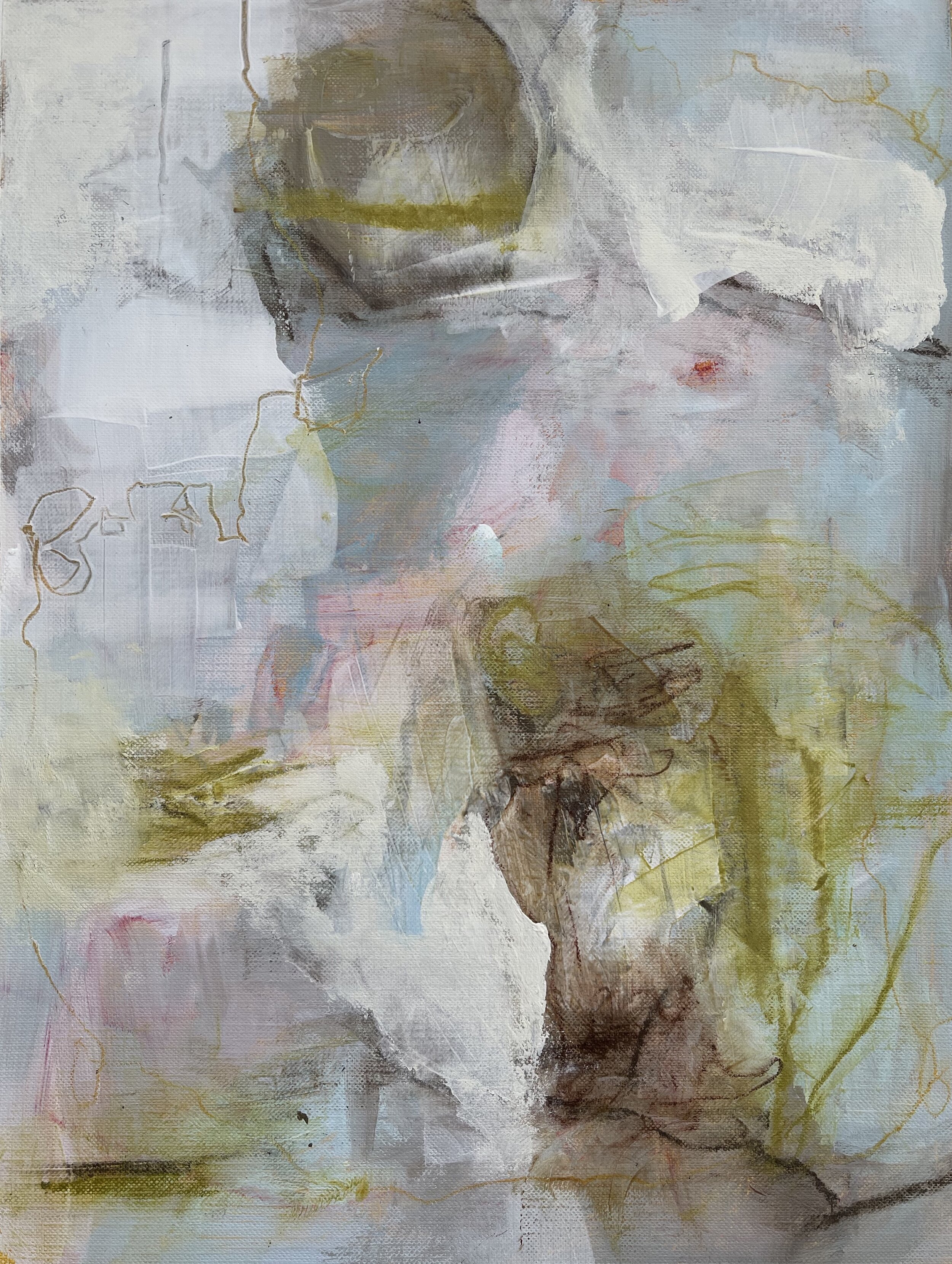This abstract painting on canvas features an intricate array of colors and textures, creating a complex and visually stimulating piece. Dominated by white, muted gold, brown, and soft red tones, the painting also incorporates hints of blue, green, and pink. The primary focus is on large, bold brush strokes that crisscross randomly and smaller, meticulous strokes that add subtle details and depth.

In the bottom left corner, a faint red streak extends toward the middle and the upper right, blending with the ambient white and gold, giving it a slightly grayish hue where colors meld. The upper middle section showcases a prominent round brown shape with scattered patches of faded white, beneath which lies a splash of light blue. This central portion also includes streaks of greens and sporadic pink lines, along with a conspicuous olive-colored stripe near the top.

A semi-circle of brown with golden lines cuts across the canvas, complemented by a faint, shadowy figure that seems to be off-center to the left, overshadowed by a white blob situated nearby. This blob overlaps and blends into brown lines that rise from the bottom right corner, where further scribbles in dark brownish-yellow cascade upward.

The painting is noticeably textured, with the rough surface of the canvas peeking through the layers of paint. Its random, messy brushwork and lack of a defined subject evoke a deeply abstract and modern artistic expression. Some viewers might discern the semblance of facial features, such as an eye and mouth toward the bottom right corner, which add an intriguing layer of interpretative potential to this otherwise chaotic composition.